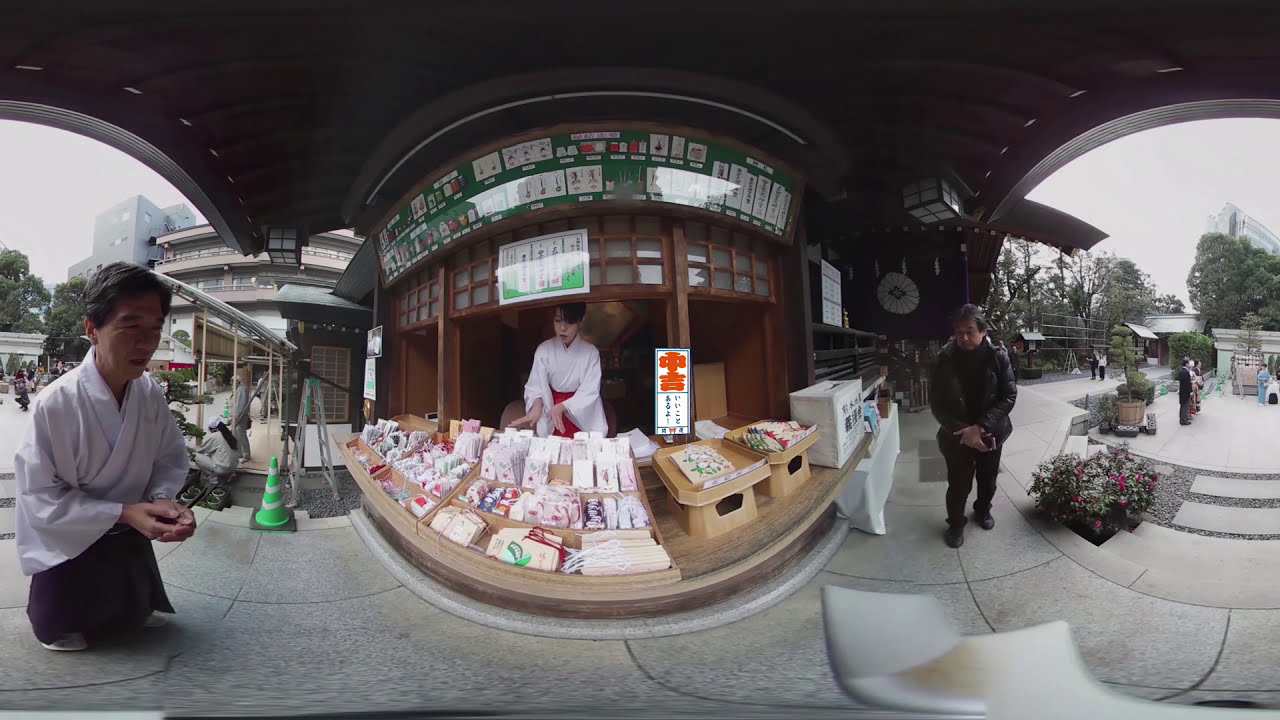This 360-degree photo captures a vibrant, bustling Asian marketplace, possibly located in Japan or China. At the center of the image is a wooden storefront, likely a bakery stand, where a woman dressed in a traditional white kimono with a red sash is selling various pastries neatly displayed in front of her. Above her head, there's a green sign listing the items for sale. To her right stands a man clad in dark clothing and a jacket, his arms crossed, holding a phone, and positioned next to a flower pot on the ground. On the left side of the image, another man is seen wearing a distinctive white and black traditional Chinese gown, standing near a green striped traffic cone and a ladder. The marketplace scene is set against a backdrop of additional buildings, trees, and indistinct shoppers, creating a lively and immersive atmosphere. The ground is paved with light gray stone, adding to the authentic feel of this Asian marketplace. The spherical distortion of the photo accentuates the central figures while giving a unique, rounded perspective to the bustling environment around them.